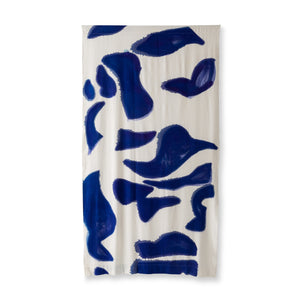The image showcases a small, professional photograph of a product, likely a towel, displayed vertically against a white background. The white fabric is slightly relaxed, creating subtle ripples and grey-edged lines that run top to bottom. A series of dark blue, abstract shapes are scattered across the towel in equal parts of large and small sizes, totaling approximately 16. Some of the blue shapes bear a slight resemblance to familiar objects, such as hats, tampons, and duck beaks. The image highlights these solid blue splotches with hints of light blue outlines against the white background, making for a striking and artistic presentation. This promotional photo could potentially be intended for a retail website or store like Target or Marshalls.